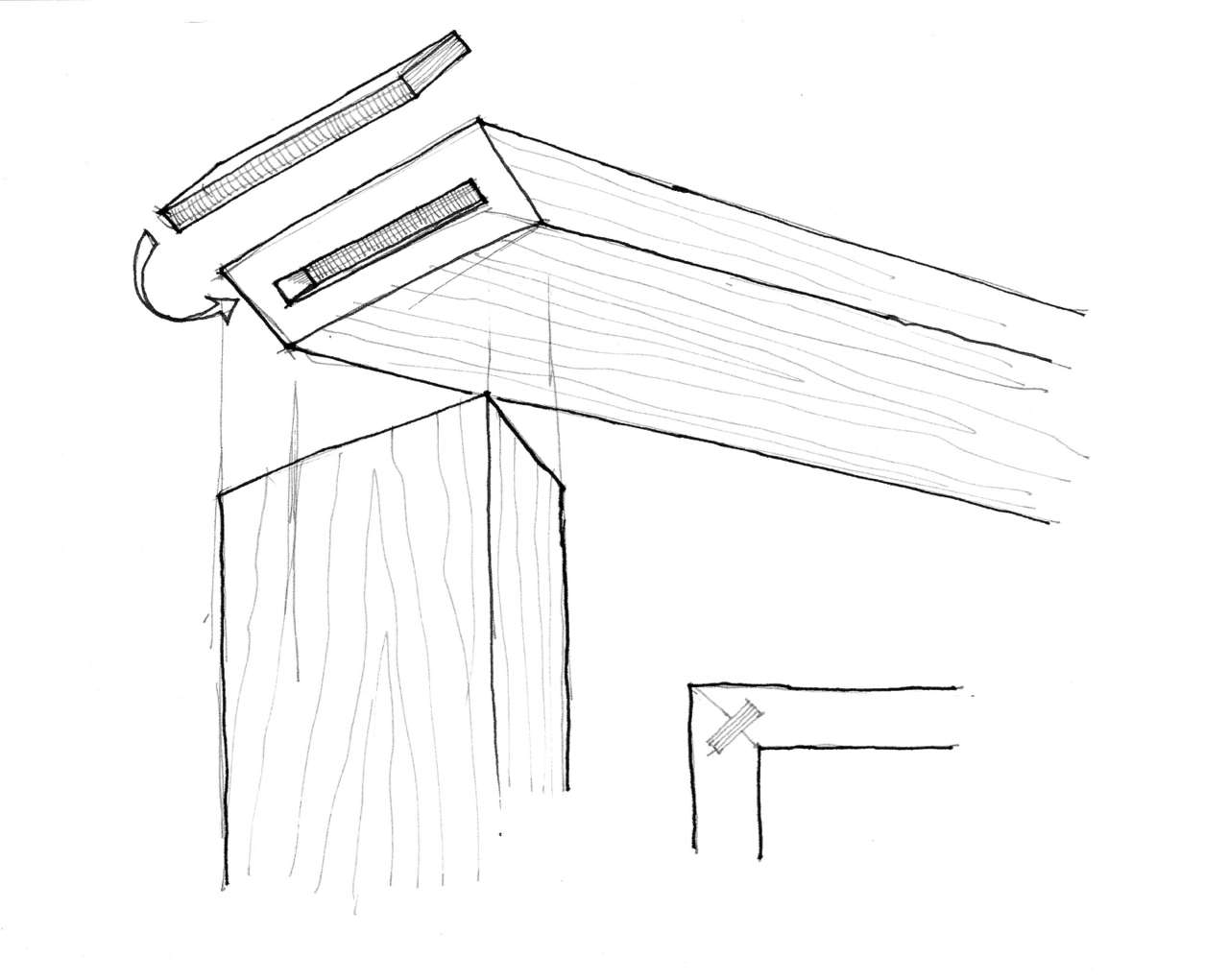This image is a simple black and white sketch with no border or background, emphasizing a wooden structure being assembled or disassembled. In the far upper left corner, there is a vertically-oriented plank of wood with detailed grain, marked with lines indicating its texture. An arrow points from this plank to a slot in a second piece, which appears to be a 2x4 piece of wood, perfectly notched to accommodate the top piece. Below this, there is another horizontal 2x4 piece of wood, similarly detailed with wood grain. The lower right corner features an incomplete frame made of two plain white boards, clearly connected at a seam, seemingly held together with a strip of tape. The arrow and the precise fit of the notches suggest this drawing is a technical plan, possibly engineered to show how the pieces should interconnect, focusing on the assembly process.